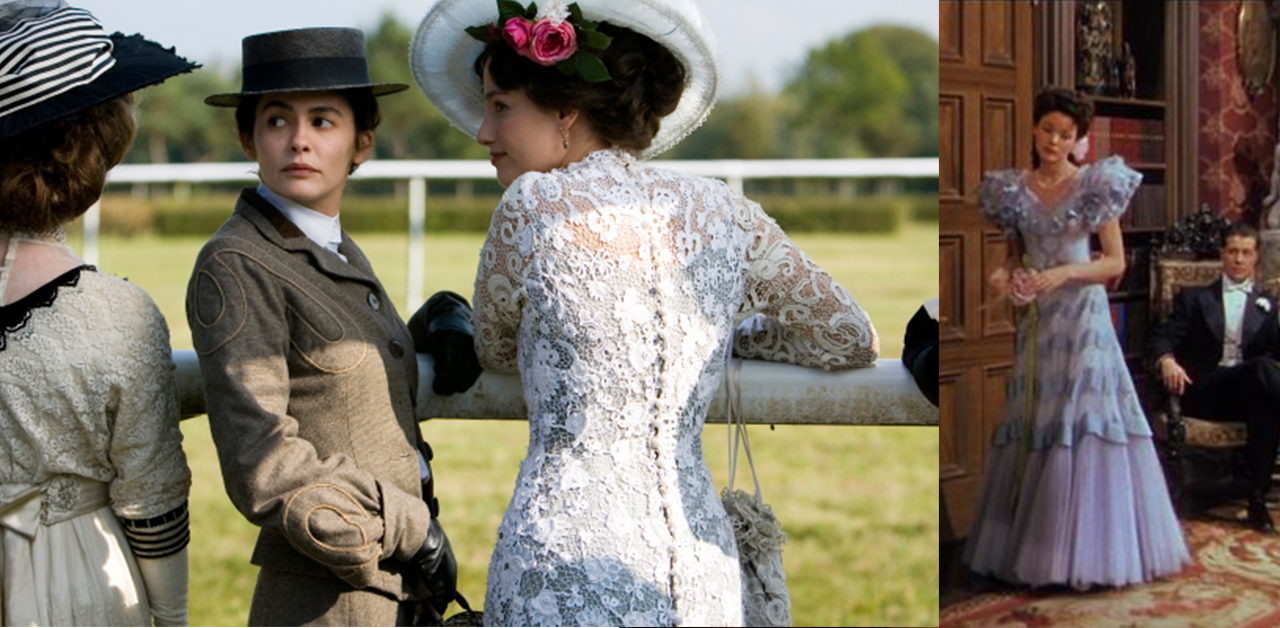A set of two images from "Coco Avant Chanel" displays an elegantly dressed group of individuals. On the left side, three women stand outdoors in front of a fence post. The first woman, in a white dress with a black undershirt, is adorned with a hat featuring white and black stripes. Next to her, another woman, wearing brown attire and black gloves, sports a small top hat and a white undershirt. The third woman, dressed in a lace dress paired with an ornate white hat decorated with roses below the brim, completes the trio. On the right side, an indoor scene is depicted with a gentleman seated in a stately, upright chair and a woman standing beside him in a floor-length gown, notable for its frilly shoulders. The elegance and detail in their attire suggest a vintage, high-society ambiance.